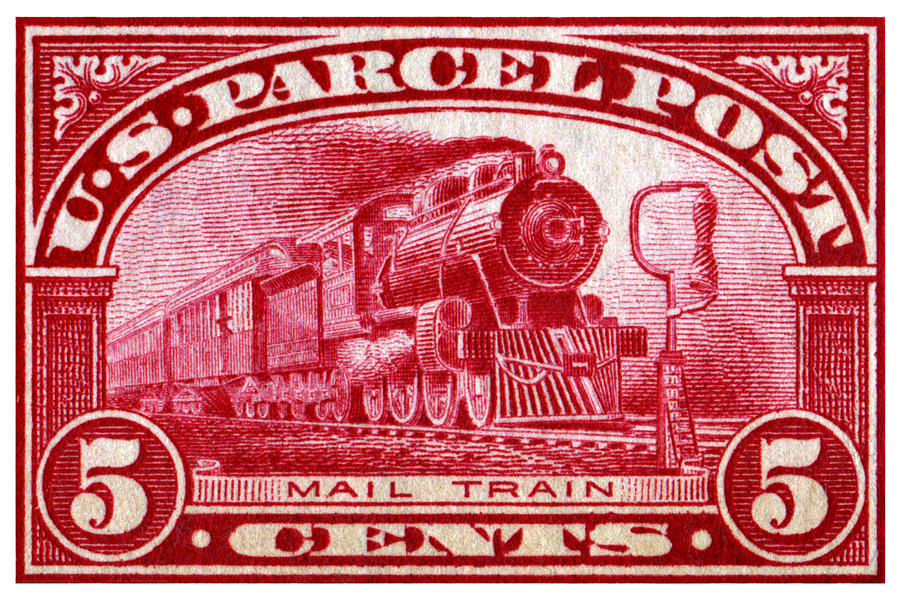The image is a detailed, blown-up portrayal of a vintage U.S. Parcel Post stamp, predominantly featuring a red and white color scheme. At the very top of the stamp, large white letters spell out "U.S. Parcel Post," framed by an intricate, stippled border with scroll tassels in the top corners. The center of the stamp showcases a steam-powered locomotive barreling down the tracks, reminiscent of early 20th-century trains. This detailed illustration includes a man leaning out of the engine window, steam billowing from the locomotive, and a coal cart followed by two passenger cars trailing behind. The train is depicted at a junction, adding to the sense of motion and industrial prowess.

The stamp is carefully designed with various bordered sections: a red outer border, a subsequent white inner border, and an arch-shaped red-and-white-striped motif housing the central image of the train. Flanking the train image are the numbers "5" in bold white, both on the left and right sides, within white-bordered red circles. Directly below the train graphic, a white banner with red letters reads "Mail Train," and beneath this, the word "cents" is displayed in smaller white letters, tying together the postage value of "5 cents." The meticulous design and historical elements suggest it is an early 20th-century postal artifact.